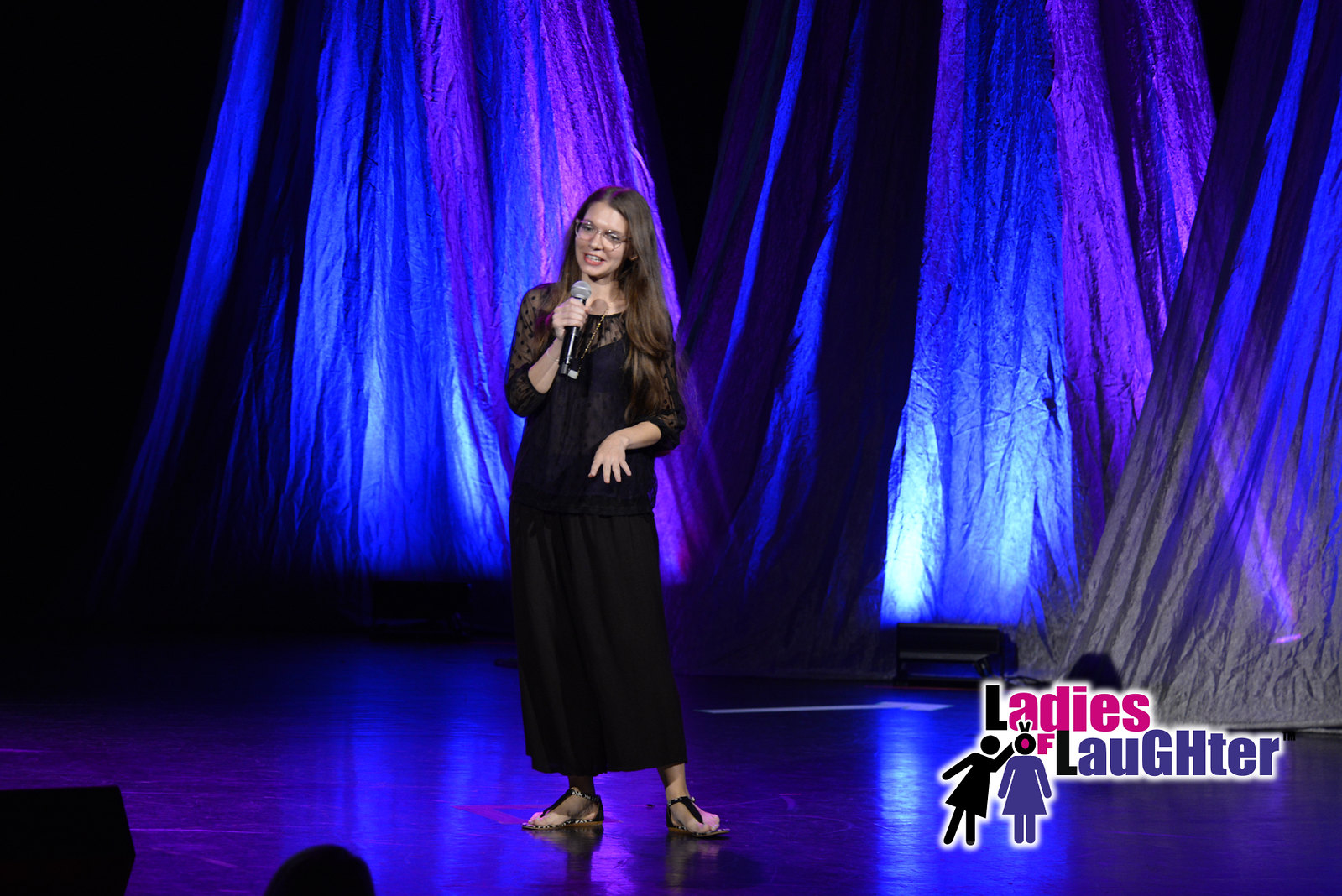In an indoor nightclub setting, an image reveals a comedian performing under vibrant, iridescent lighting. The backdrop consists of blue and purple illuminated curtains. At the forefront stands a Caucasian woman with long, dark brown hair cascading down to her mid-back. Dressed in a long-sleeved, sheer, black dress and sandals, she holds a black microphone with a gray top, speaking animatedly. She wears glasses and extends one hand expressively forward. The image captures the ambiance with subtle hints of the audience, notably a head visible at the stage's front. In the bottom right corner, a logo reads "Ladies of Laughter," accompanied by two stick-figure icons of women, one in black and the other in purple, creating a playful interaction. Two indistinct black objects lie at the stage's bottom left, shrouded in mystery.